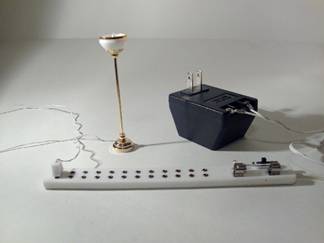This is a detailed photograph of various electrical items placed on a white surface, with a white wall serving as the background. Central to the image is a long, rectangular, white extension cable or circuit board. Attached to this extension is a small white device with a wire connected to it. Situated next to this device is a black European two-pin plug, which is positioned upright, revealing its two prongs and a duo of extending wires. Near the extension cable, there is a golden brass lamp with an unlit bulb and a white shade, which is slightly taller than the small connected device. The lamp's wires extend from the end of the extension cable toward it, cascading outwards. The careful arrangement casts subtle shadows on the white background, showcasing the intricate wiring and placement of each object in the composition.